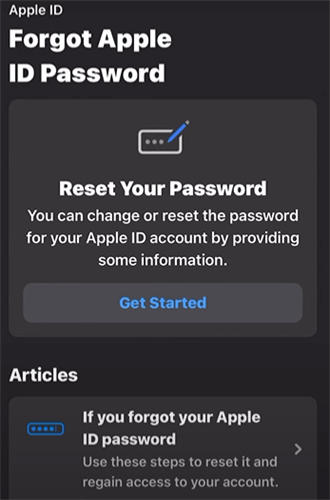This screenshot showcases a section of the Apple ID password recovery page. Dominated by a sleek black background, large white text prominently declares, "Forgot Apple ID password." Below this, the page illustrates a process with an image featuring three dots, a crayon, and a box, emphasizing the capability to "Reset your password."

The detailed instructions indicate that you can change or reset your Apple ID password by providing some necessary information. A clickable box labeled "Get Started" invites users to begin the process. Beneath this, an additional informational segment includes white text detailing, "If you forgot your Apple ID password, use these steps to reset and regain access to your account." Adjacent to this statement is an image of a rectangle containing four blue dots.

No further visible steps are included in the screenshot as the page appears to be cut off, suggesting that more information would be available upon scrolling. The overall design is minimalistic and straightforward, focusing attention on the primary actions with contrasting blue elements and strategically placed graphics.